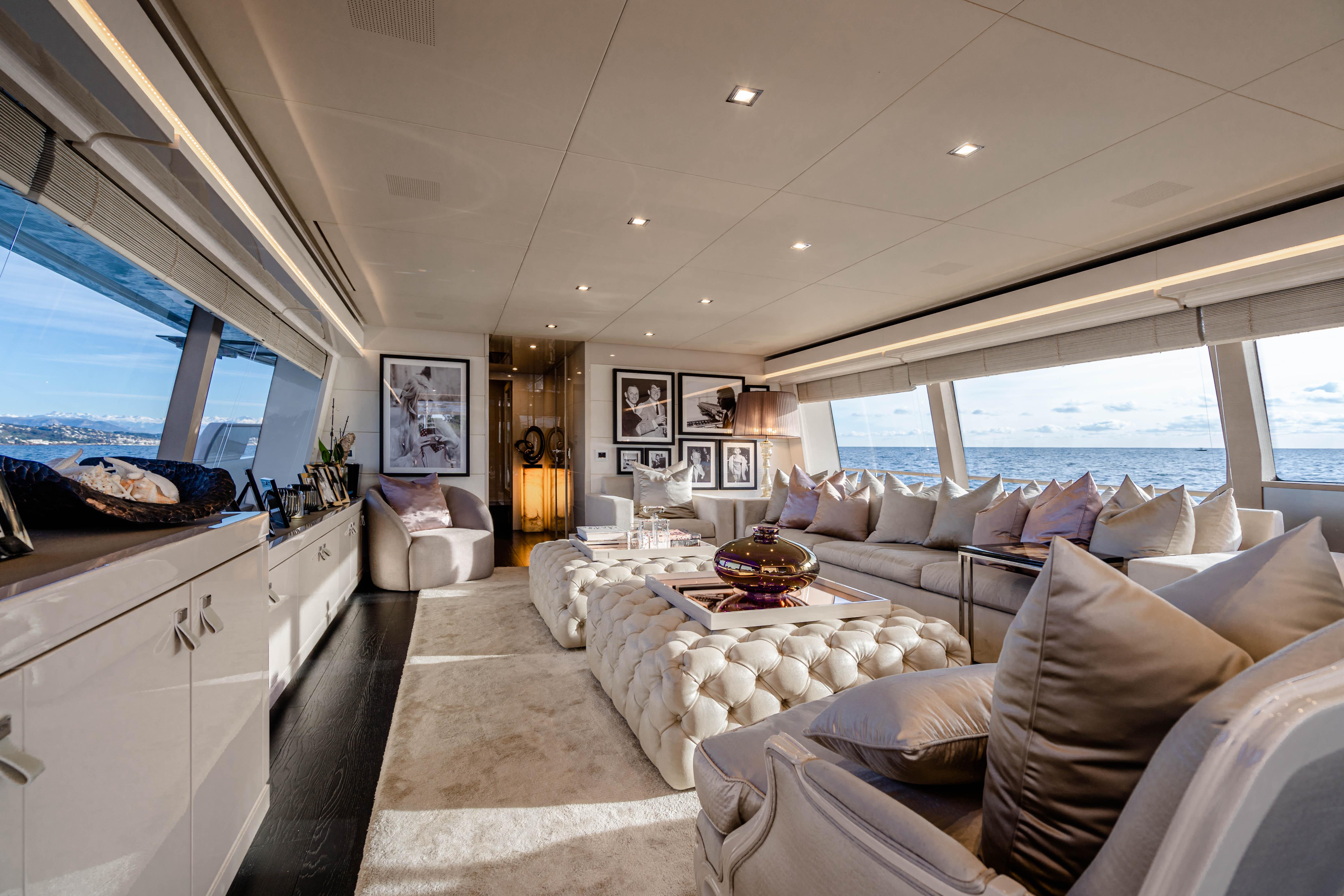This photograph captures the luxurious interior of a high-end yacht. The space is a plush, elongated room adorned with elegant and opulent décor. Both sides of the room feature expansive windows showcasing serene waters—on the right, only the water is visible, while the left window offers a glimpse of a distant island or landmass.

On the left side, there’s a series of white cabinets with handles, and on top of the closest countertop sits a black shell-shaped artwork holding smaller white shells. Further down, a lower counter is decorated with picture frames and floral greenery. Beyond this, in the far top left corner, there’s a rounded chair on the floor, adorned with a silk square pillow, positioned by a large black-and-white photograph of a woman holding an enigmatic object. 

The back wall is a gallery of seven framed photographs, two of which are poster-sized. One features two men in suits smiling at the camera, and the other shows a man in profile with a background hinting at a bridge or wharf. Below these are smaller photos, yet their details are less discernible. Beneath the gallery sits a square chair with two pillows next to a prominent lamp.

The right side of the room is dominated by a sumptuous white couch enveloped in roughly a dozen pillows. In front of the couch, two plush tufted coffee tables serve as focal points; one adorned with a decanter set and the other with a decorative glass globe on a square serving tray. A fluffy chair with three pillows is nestled at the end of the couch, adding to the lavish seating arrangement.

The dark plank wooden flooring grounds the room’s design, overlaid with a creamy white rug that nearly covers the entire room. The ceiling, like much of the interior, is a pristine white, punctuated by strips of lighting that lead down the center, creating a bright and inviting ambiance befitting such a sophisticated yacht.